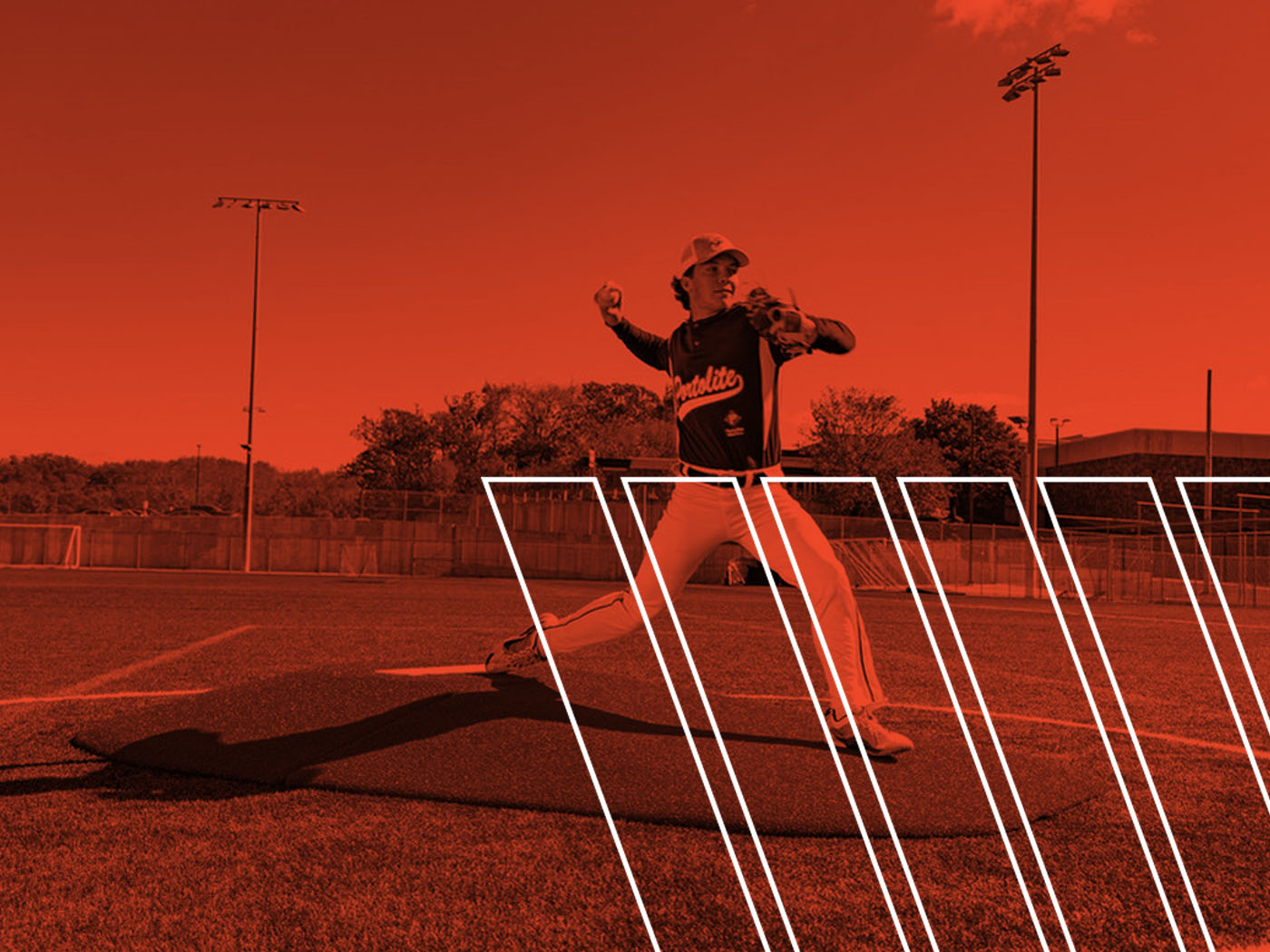The image captures a teenage pitcher, possibly from a high school or amateur league, in mid-pitch on a baseball mound. The photograph is heavily edited with a deep red filter that engulfs the entire scene, creating a dramatic tone. The pitcher, wearing white pants and a darker top – possibly with "Charlotte" written on it – is right-handed and appears to be in the act of releasing a baseball. His profile angle towards the camera accentuates his focused expression and poised form. The backdrop features tall stadium lights and a wooden fence with trees beyond, indicating a typical baseball field setting rather than a large stadium. Notably, the photo includes a series of five abstract white rectangles diagonally superimposed on the lower right corner, adding an artistic element to the composition.